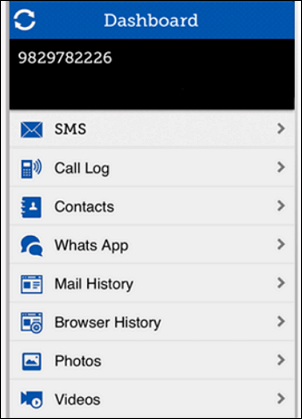At the top of the image, there is a blue banner that spans across, with the word "Dashboard" prominently displayed in white text. Below this banner, the central section features a black box with white numbers reading "982-978-2226." Surrounding this box, the remainder of the page is gray and organized into various categories listed vertically.

- The first line has a blue envelope icon accompanying the label "SMS" in black text and a gray arrow on the far right.
- The second line features a blue cell phone icon next to "Call Log" in black text, also with a gray arrow on the right edge.
- The third line includes a blue address book icon beside the word "Contacts," again with a gray arrow to the right.
- This pattern continues with subsequent lines labeled "WhatsApp," "Mail History" (with a blue envelope icon), "Browser History," "Photos" (with a blue photo icon), and "Videos" (with a blue video camera icon), each accompanied by a gray arrow on the right side of the line.

The overall layout is clean, with clear categories and icons for easy navigation, emphasizing a user-friendly dashboard interface.